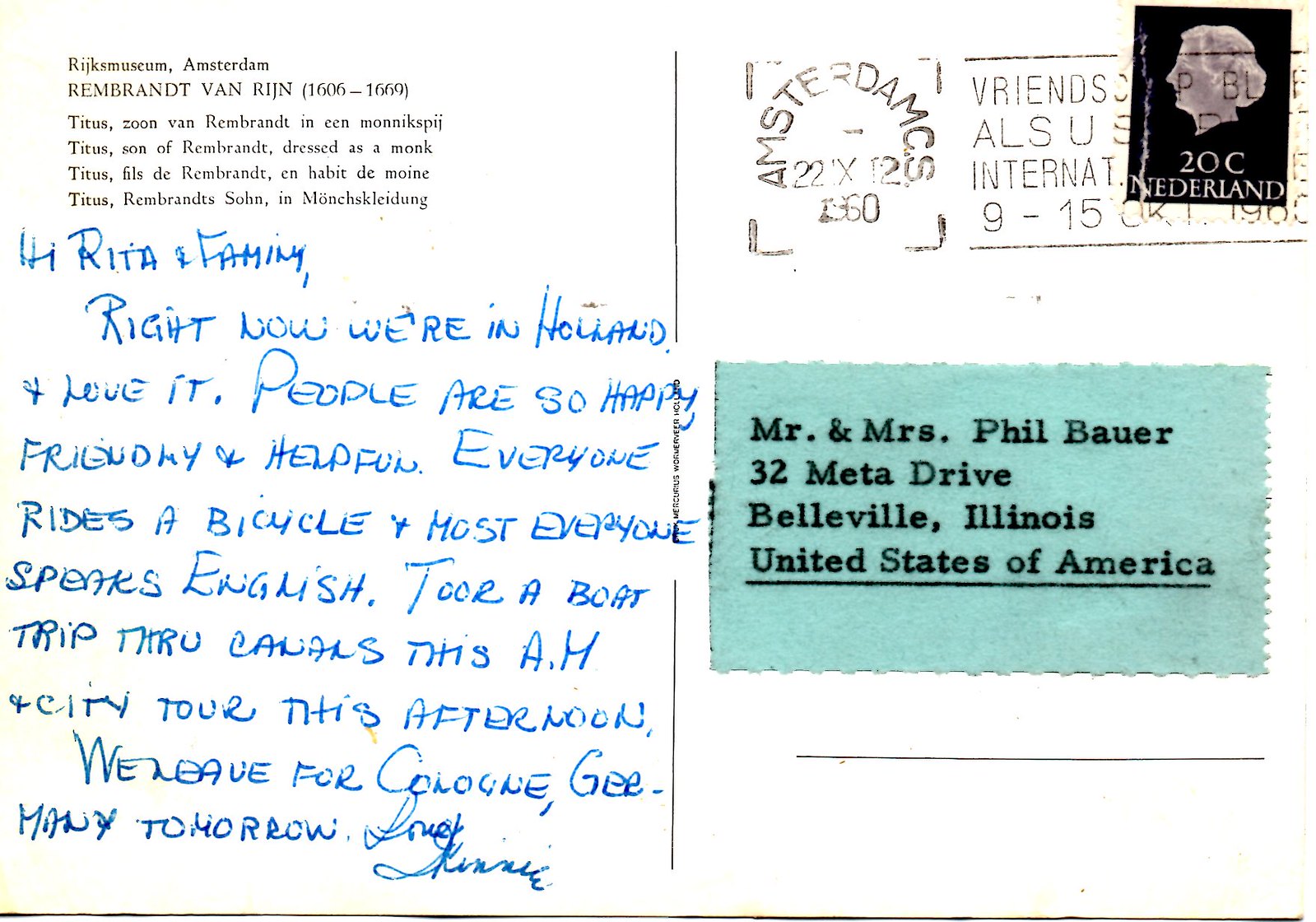This image captures a postcard addressed to Mr. and Mrs. Phil Bauer at 32 Meta Drive, Belleville, Illinois, United States of America. The postcard, predominantly white with a green rectangular highlight, holds a handwritten message in blue ink. The sender, currently in Amsterdam, shares their joy about being in Holland, mentioning that people are happy, friendly, and helpful. They observe that almost everyone speaks English and rides bicycles. They recount their morning boat trip through the canals and a city tour in the afternoon, noting their departure to Cologne, Germany the next day. 

In the upper left corner, there's an address and a reference to the Rijksmuseum and Rembrandt van Rijn (1606-1669). A 20-cent black stamp featuring a bust is located in the upper right-hand corner, with a postmark above it stating “Amsterdam 22-12.” The date on the postcard seems to be September 15, 1960. The message concludes with the sender’s love, though the signature is illegible.